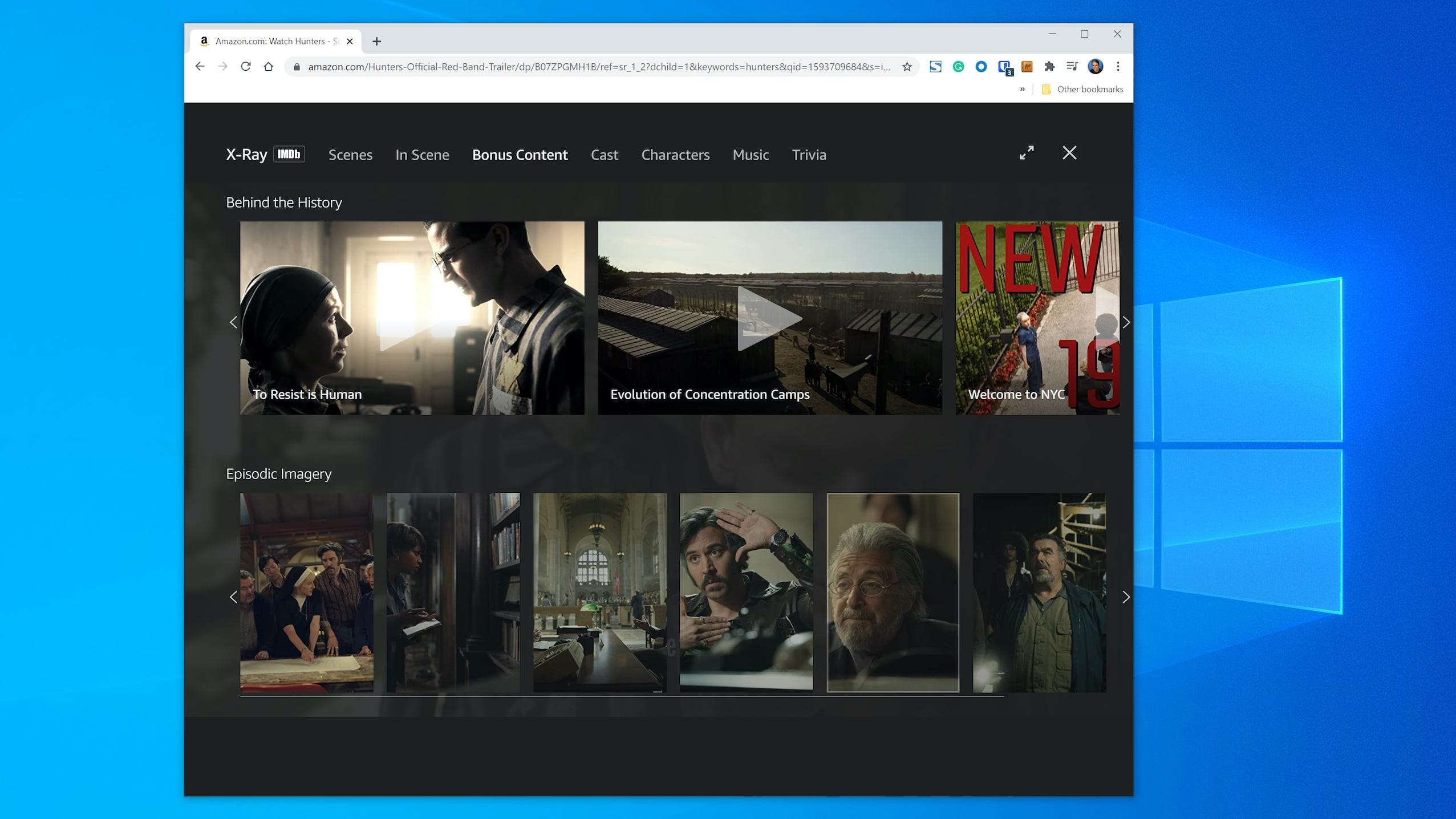The image is a screen capture of a web page showcasing a video page dedicated to the official Red Band trailer of the film "Hunters" on Amazon.com. The background of the page is completely black, and the top ribbon displays several elements. To the very upper left, it says "X-Ray" followed by "IMDb," with various tabs to the right labeled Scenes, In-Scene, Bonus Content, Cast, Character, Music, and Trivia. The Bonus Content tab is currently selected.

The main field of the page is divided into two main sections. The first row, titled "Behind the History," contains three thumbnail images. The first image is labeled "To Resist is Human," the middle image is labeled "Evolution of Concentration Camps," and the third image is titled "Welcome to New York."

The bottom section, labeled "Episodic Imagery," appears to display a series of images that likely follow a sequential order, presumably extracted from the film.

At the very top of the screen capture, the web address bar is visible, clearly indicating the URL "amazon.com hunters official red band trailer," specifying that the page belongs to the official Red Band trailer for the movie "Hunters."

This detailed screen capture displays various in-depth content and features available for the film, emphasizing its historical and narrative elements through its bonus content and episodic imagery.